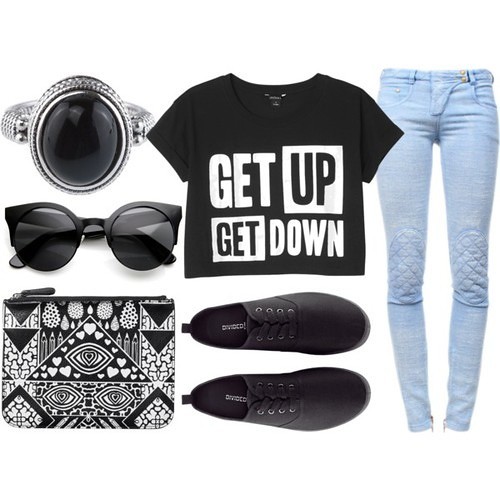This image displays a collection of accessories and clothing items set against a stark white background, likely for a product listing. In the upper left corner, there's a silver ring featuring a large, dark, shiny gem reminiscent of a mood ring. Just below the ring, a pair of rounded, dark-rimmed sunglasses are positioned. To the left of the center, a black and white cosmetic bag adorned with illustrations of triangles, hearts, and eyes adds a stylish touch. 

At the top center of the image, a black t-shirt boldly displays the text "Get Up, Get Down." Below the t-shirt, a pair of black shoes with indiscernible branding are turned slightly towards the right. Finally, on the far right of the image, a pair of light blue jeans completes the ensemble. This array of items collectively highlights a casual yet trendy mix of fashion accessories and apparel.